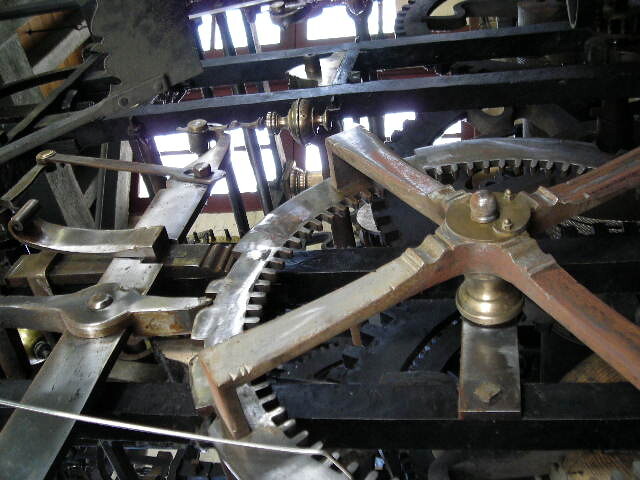This close-up photograph showcases the intricate inner workings of a large piece of machinery. Dominating the image is a substantial silver-colored round gear, adorned with a reddish rusted metallic X-shape overlay. This main gear's inner core is brass, featuring a brass nut at the top. Encircling this main component, numerous black gears and cranks interlock, orchestrating complex movements.

The upper section of the large gear is intersected by two horizontal iron bars. To the left, a vertically oriented iron bar supports three medium-sized horizontal bars, extending toward another bar. Surrounding the central gear, an array of silver bars, cylindrical components, and scaffold structures—varying from black to dark and light gray—create a web of interconnecting parts.

To the left side, a series of silver pieces form bars and cylindrical components, some resembling shears gripping the adjacent rotating gear. Additional scaffolding above adds to the complexity, casting shadows and adding depth. Behind the machinery, a concrete wall serves as a stark backdrop, with light filtering from above, illuminating the scene in a soft glow. This detailed depiction captures the impressive scale and precise engineering of the intricate machine workings.